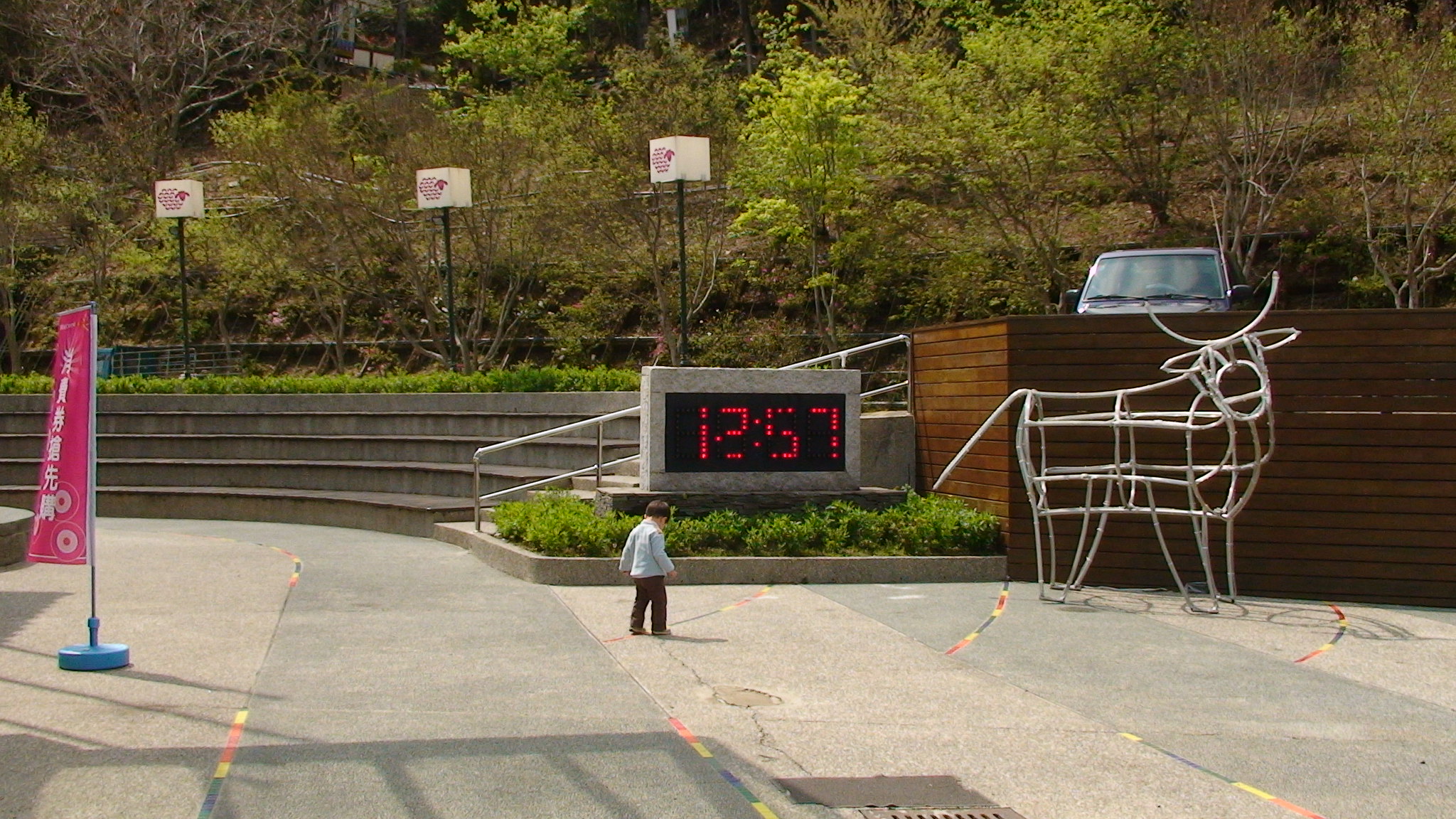In this photograph, a young boy, likely around two or three years old, wanders alone in a spacious outdoor area likely near a tourist attraction or public building. The child, dressed in a blue jacket and brown pants, is engrossed in inspecting the cracks on the concrete pavement. Prominently, a large digital clock displaying the time '12:57' with several burnt-out red lights set against a black background serves as a focal point ahead of him. This clock is framed by a flight of concrete stairs with metal handrails and is bordered by lush bushes. Directly behind the boy, approximately ten feet away, a flag featuring Asian characters, red in color with a blue pole, suggests a cultural or celebratory context. Additionally, an artistic metal sculpture resembling a moose, comprised of metal pipes, stands to his right, adding to the artistic ambiance of the scene. This setting, which includes stone and marble-like features, multiple light posts, and extensive concrete areas, hints that this might be an establishment like a museum or an urban park. Trees and a wood wall enclosing a parking lot can be seen in the background, contributing to the secluded yet open environment.